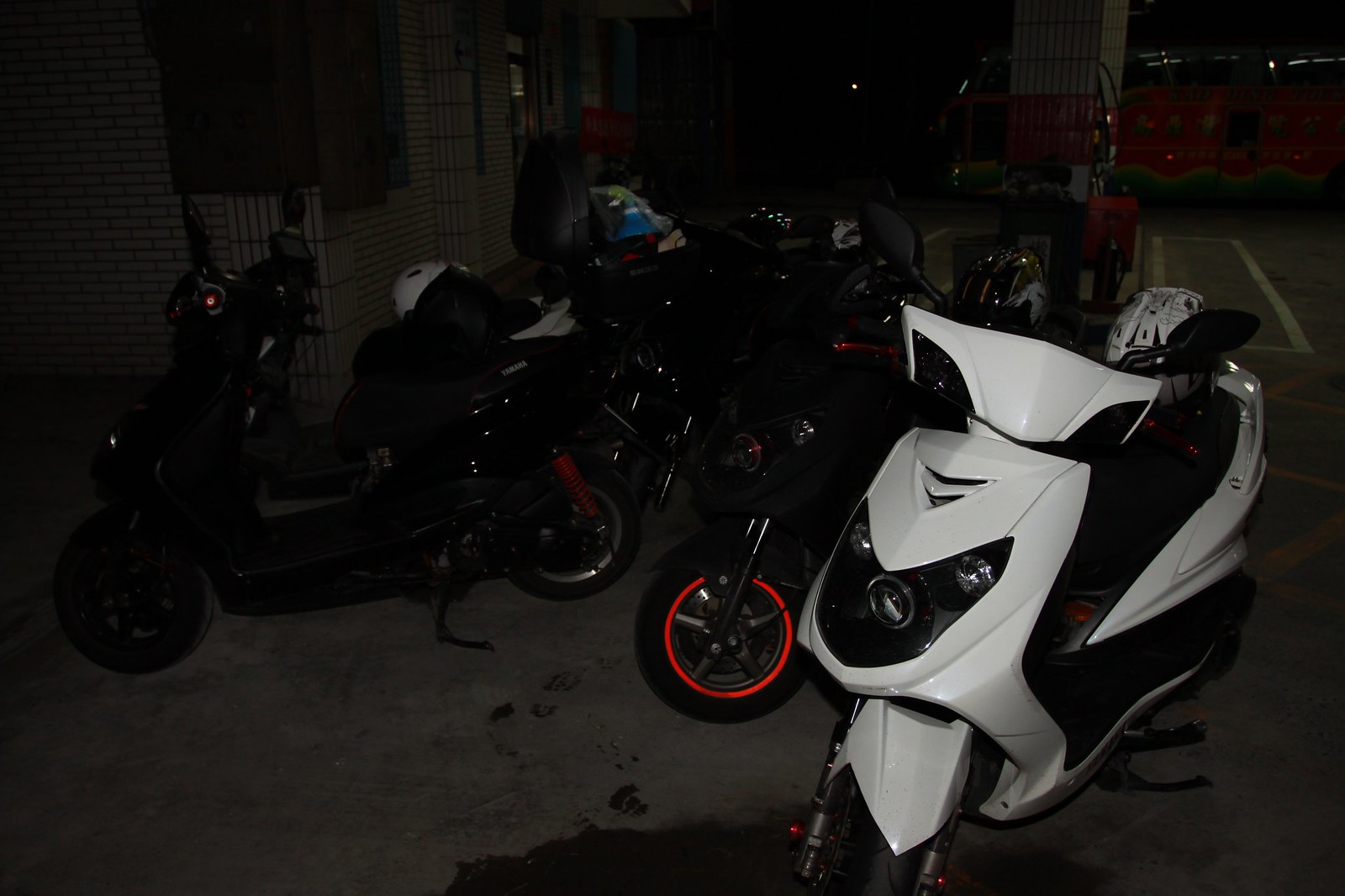This nighttime photograph, cloaked in darkness and an eerie foreboding atmosphere, captures a street scene with a series of motorcycles positioned in what appears to be a parking lot. Dominating the frame is a black and white motorcycle closest to the camera, distinguished by a white helmet perched on its back. While the lack of lighting makes it difficult to discern details, another notable motorcycle features a striking red stripe on its front wheel. Most of the motorcycles appear to be black or dark in color, blending into the dimly lit surroundings. In the backdrop, a light gray brick building is faintly visible in the upper left corner, adding a sense of structure to the overall dark and shadowy environment.